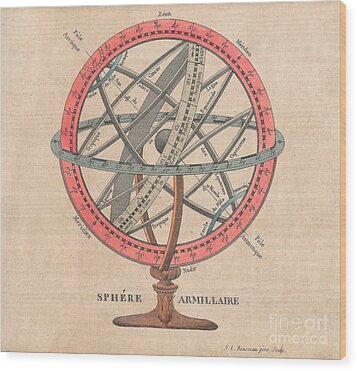The image depicts a detailed painting of a historical armillary sphere, presented as a flattened, two-dimensional drawing or print on a light brown wooden plaque. The wooden background is characterized by horizontal lines that emphasize the grain. Central to the composition is the sphere, which is mounted on an elongated brown stand. The sphere features a prominent dark pink circle on the outside, with additional interconnected circles inside, varying in shades of silver and gray. These circles represent latitude, longitude, and meridian lines, intricately intersecting in a globe-like arrangement. Although the numbers and measurements on the circles are too small to discern, they add to the scientific and decorative detail of the piece.

Written on the base in black print are the words "Sphere Amillare," likely referring to the term "armillary sphere," an ancient astronomical instrument. The painting is signed at the bottom, though the signature is illegible, and a watermark in the bottom right corner reads "Fine Art America." The overall effect is a meticulous representation of a scientific illustration, blending artistic elements with historical educational value.